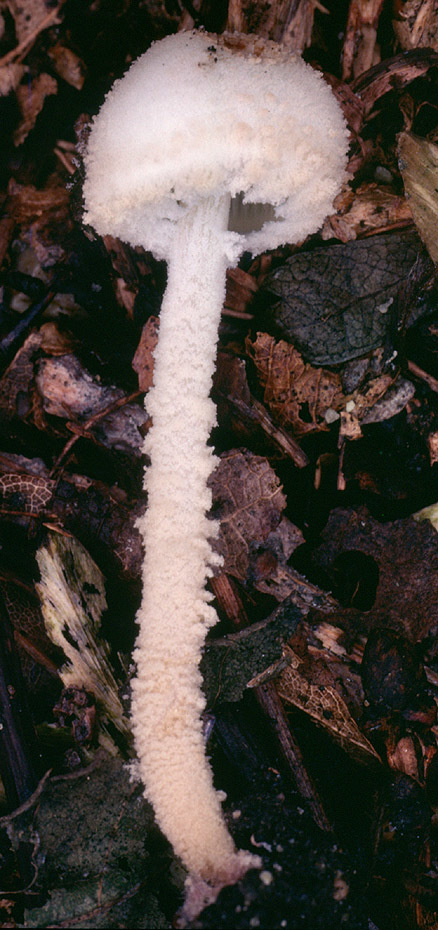This vertically aligned, rectangular image showcases a decaying, fuzzy white toadstool, prominently centered on a forest floor strewn with wet, brown leaf litter and decomposed wood. The mushroom, resembling grated cheese in texture, has a relatively long stem — approximately 3 inches — and a smaller cap around 2 inches in diameter. Brownish streaks and a distinctive brown spot mark the otherwise snowy white cap, adding contrast to the fuzzy appearance that extends down the entire length of the stem. The background's dark earthy tones enhance the visibility of the gray underside of the cap and the striking white of the toadstool, highlighting its decaying yet striking presence amid the forest debris.